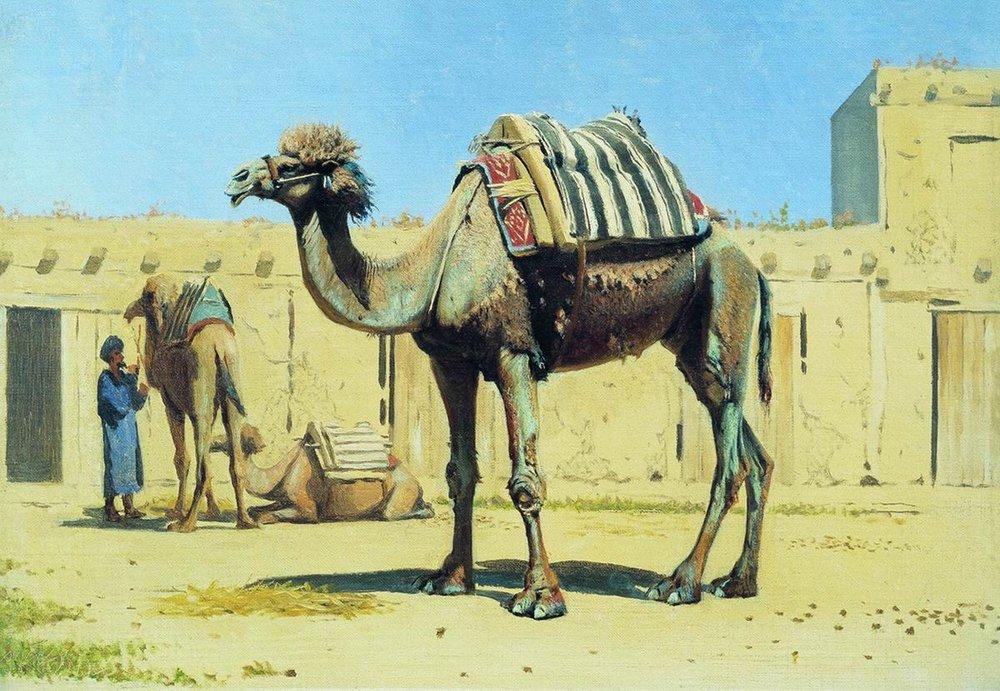This painting depicts a detailed and surreal realist scene centered around three camels in a Middle Eastern setting. The most prominent camel in the foreground sports a spiky mane and bears a padded load that resembles a mattress. Rich turquoise hues adorn its skin, lending a surreal touch to its realistic form. To the left, a man dressed in a traditional long robe and headdress tends to a second camel, guiding it by its ropes. This camel stands adjacent to a small two-story clay building that accents the sandy, tan, and light brown tones dominating the backdrop. A third camel reclines on its knees and elbows nearby. The scene is set against what appears to be a castle or similar structure, characterized by its tan and brown colors, evoking an arid, desert environment with minimal vegetation. The artist’s use of color includes touches of green, yellow, white, blue, black, and red, subtly enriching the composition.